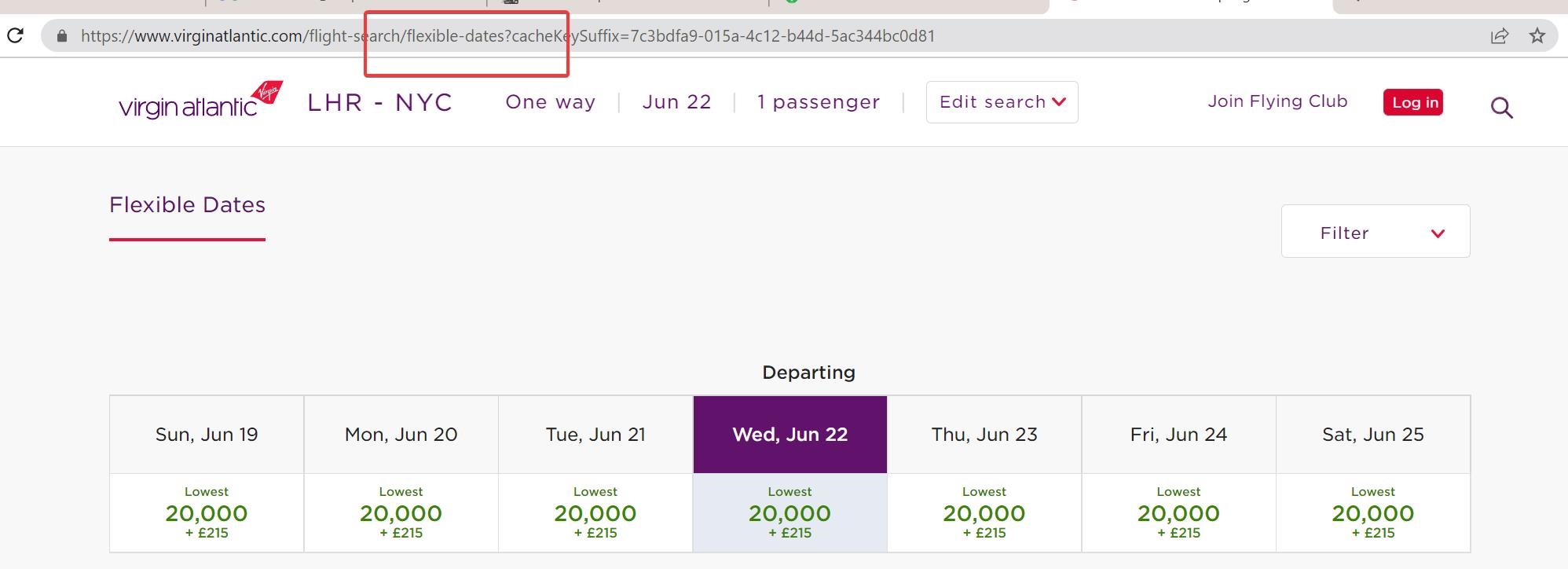Screenshot of a flight search results page on the Virgin Atlantic website for a one-way flight from London Heathrow (LHR) to New York City (NYC) for one passenger with flexible dates. The Virgin Atlantic logo is displayed prominently at the top left corner. The search criteria is stated as LHR to NYC, one-way, June 22nd, for one passenger. Options to edit the search, join the flight club, and log in are available on the right-hand side.

The "Flexible Dates" section lists departure options from Sunday, June 19th to Saturday, June 25th. Each date box provides the lowest available points and cost, consistently showing 20,000 points plus £215 for all dates within the specified range. The interface is clean and straightforward, offering clear options for flexible date searches. This consistency in points and costs implies no variance in rewards or additional costs for the selected week.